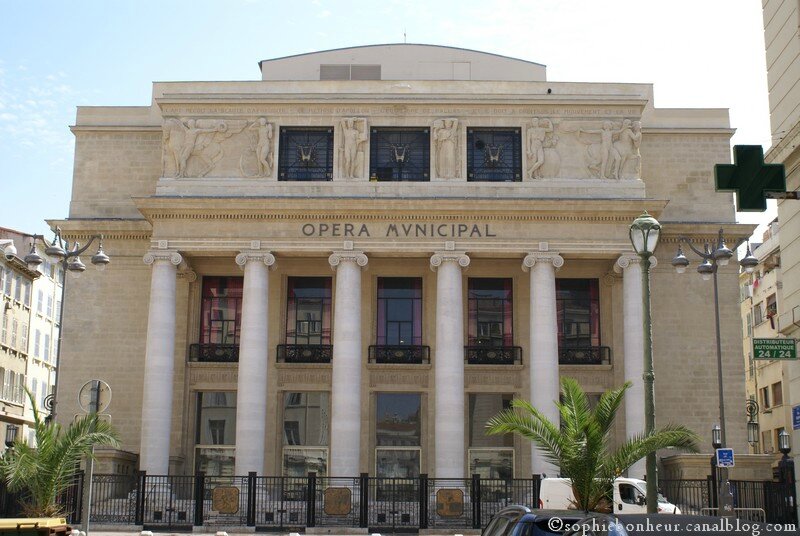The image depicts the neoclassical façade of a sprawling, tan-colored building identified as the "Opera Municipale" in bold, black lettering at the top. The sky above is a striking blue with the left side a lighter shade and the right side appearing almost white, possibly due to sunlight. The building's impressive frontage features six towering Doric columns of a concrete white hue, contrasting subtly with the lighter sandstone color of the structure. Across the top, three dark windows are adorned with base relief figures depicting human forms. Beneath these windows and behind the columns, black-framed windows and entry doors with large windows above them can be seen. A black wrought iron fence with intricate design runs along the front, accompanied by a pair of miniature palm trees—one on each side of the building. On the right side, a light post stands beside a minivan facing outward. Also visible are fragments of adjacent buildings and obscure street signs. The lower edge of the photograph bears a white copyright credit.